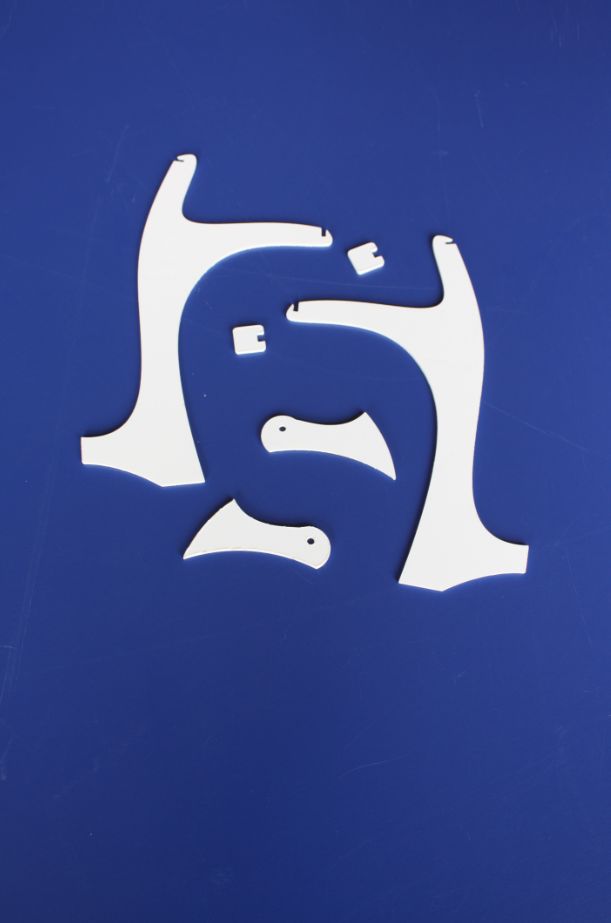The image features a vertically oriented, dark blue rectangular background with a subtle vignette effect around the edges. Overlaid on this background are six distinct white shapes arranged in an asymmetrical pattern. Prominent among these are two large, Y-shaped forms with tails, resembling deer antlers or forearms with open hands, placed near the top. Between these larger pieces are two small white squares, each marked with a tiny groove on the right-hand side. Near the bottom, nestled between the larger Y-shaped figures, are two medium-sized shapes, evoking the forms of little ghosts or fish. The intricate arrangement of these white objects against the blue backdrop creates an impression akin to a puzzle, with each piece having a unique shape and position.